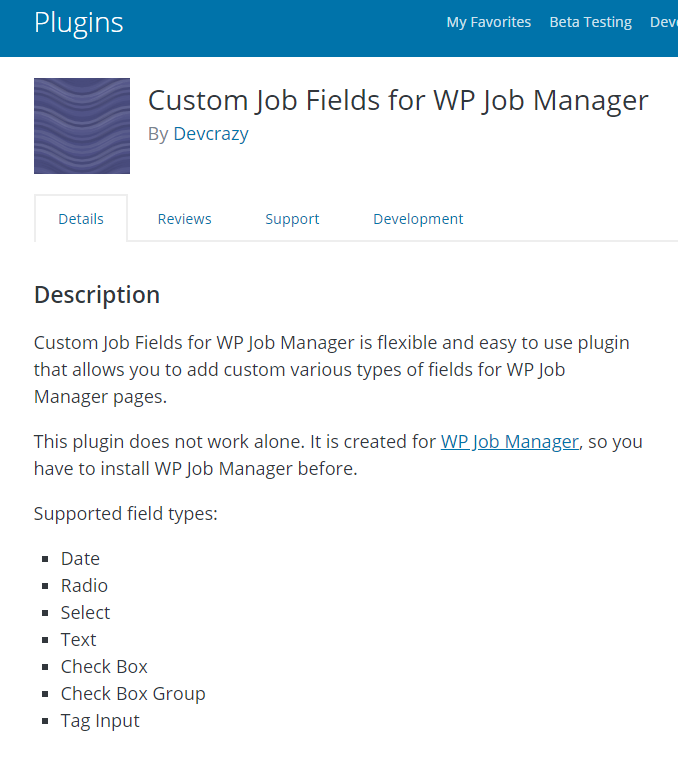The image is a screenshot of a website, showcasing a section of a plugin details page. At the top, there is a partially visible blue navigation bar containing the options: "Plugins," "My Favorites," "Beta Testing," and an abbreviation that reads "DEV," likely short for "Development." Below this bar, there is a square graphic featuring purple and black wavy lines.

The main heading on the page is "Custom Job Fields for WP Job Manager by devcrazy," with "devcrazy" being a clickable blue hyperlink. Beneath this heading are four tabs labeled "Details," "Reviews," "Support," and "Development," with the "Details" tab currently selected.

Under the "Details" section, the subheading is "Description." The accompanying text explains that "Custom Job Fields for WP Job Manager" is a flexible and easy-to-use plugin designed to add various types of custom fields to WP Job Manager pages. Important to note is that this plugin does not function independently and requires the prior installation of WP Job Manager, which is also a hyperlink.

The supported field types listed include: date, radio, select, text, checkbox, checkbox group, and tag input.